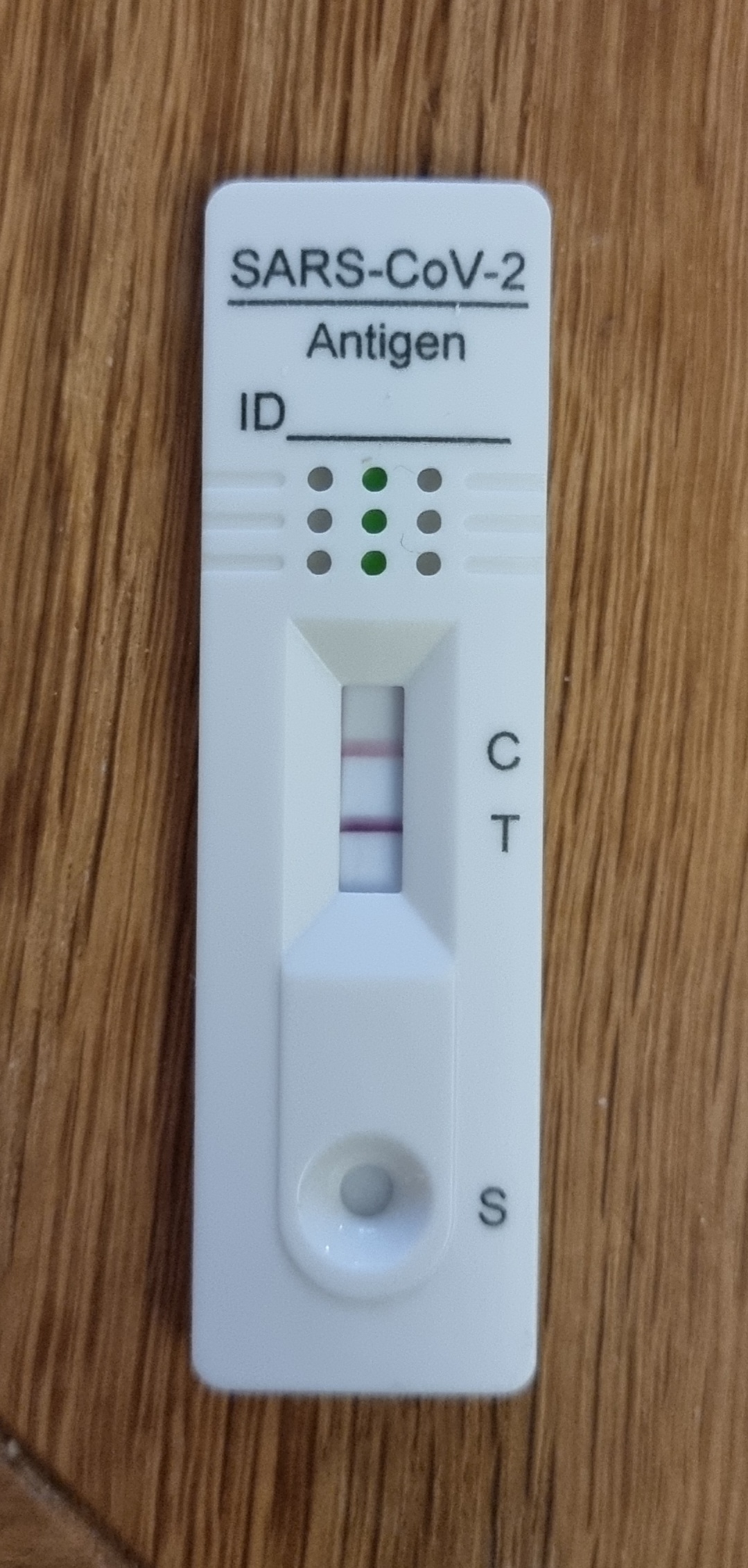The image is in a portrait orientation, featuring a device for testing SARS-CoV-2, commonly known as COVID-19. The background is a wood grain table upon which the test unit is placed. The test unit itself is rectangular and white. At the top of the unit, the text "SARS-CoV-2" is prominently displayed and underlined, with the word "antigen" written beneath it. Below this heading, there is a section labeled "ID" with a blank line next to it intended for identification purposes.

Further down, there are nine small circular dots arranged in a 3x3 grid. The dots in the center of this grid are green, while those on the outer edges are gray. Flanking the grid on either side are indented white lines. 

Below the grid is a window with indicators to the right of it: a "C" for control at the top and a "T" for test below it. Inside this window, two lines are visible: the upper line is pink and the lower line, next to the "T," is a blend of pink and purple.

At the bottom of the unit is a circular cutout with a white interior. Adjacent to this cutout is the letter "S" printed in black.